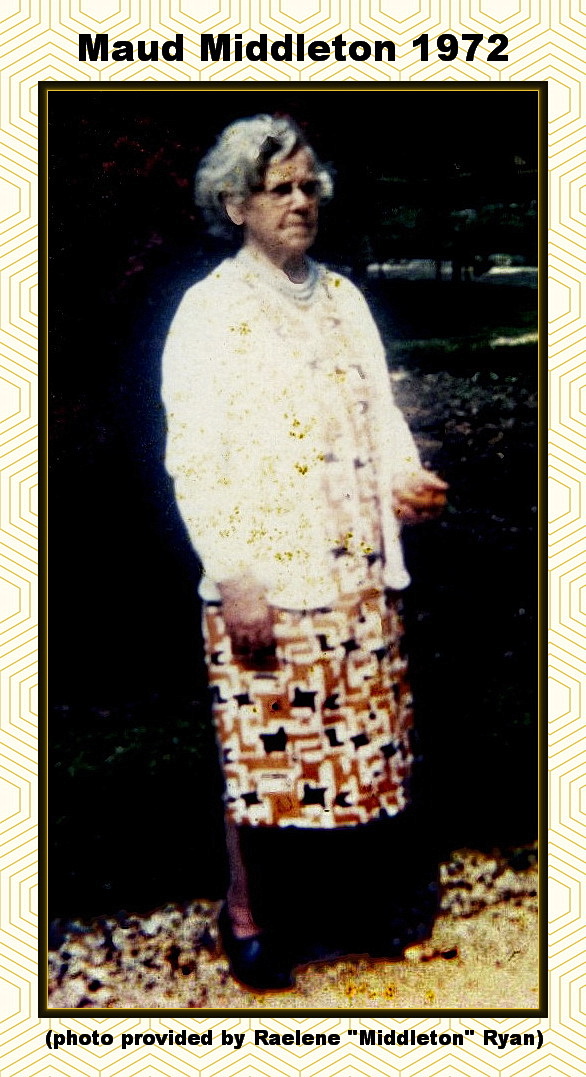This 1972 photograph, titled "Maude Middleton" in prominent black font at the top, was provided by Raylene Middleton Ryan and shows an elderly woman standing outdoors against a dim, partially obscured background. Maude Middleton, appearing to be in her late 70s or 80s, has short, curly gray hair and wears glasses. She is seen donning a white sweater or cardigan over a colorful, patterned dress featuring shades of orange, brown, black, and white. Her attire includes stockings and black, clunky shoes. The image, slightly out of focus, also hints at a yellow geometric background and possibly some trees in the distance. Maude is captured gazing to her right, adding to the serene nature of this old, cherished family photograph.